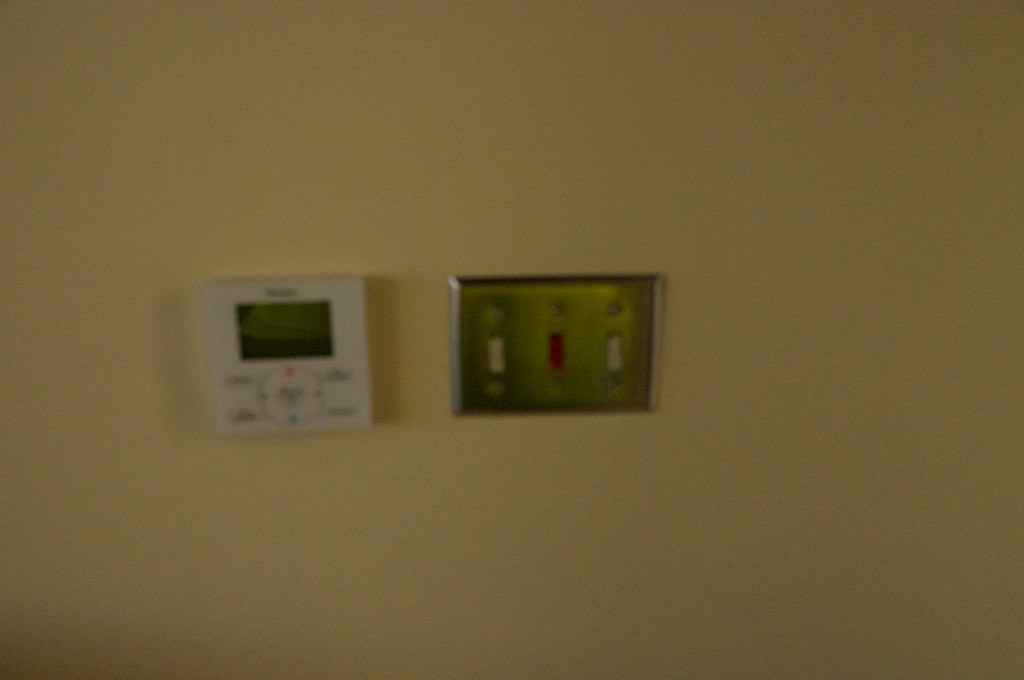In the center of a dim, blurry photograph, a tan-colored wall is partially visible, adorned with two distinct fixtures that draw the viewer's attention. On the left, a small, white, square thermostat sits unlit, its dark screen hinting at the potential for multiple settings accessible via a touch-sensitive interface. To the right of the thermostat, a brass-colored metal plate houses three light switches in a vertical arrangement. The two outermost switches are white, while the middle one stands out with its dark brown hue. The overall image is poorly lit and slightly out of focus, likely due to the movement of the person capturing the photo.